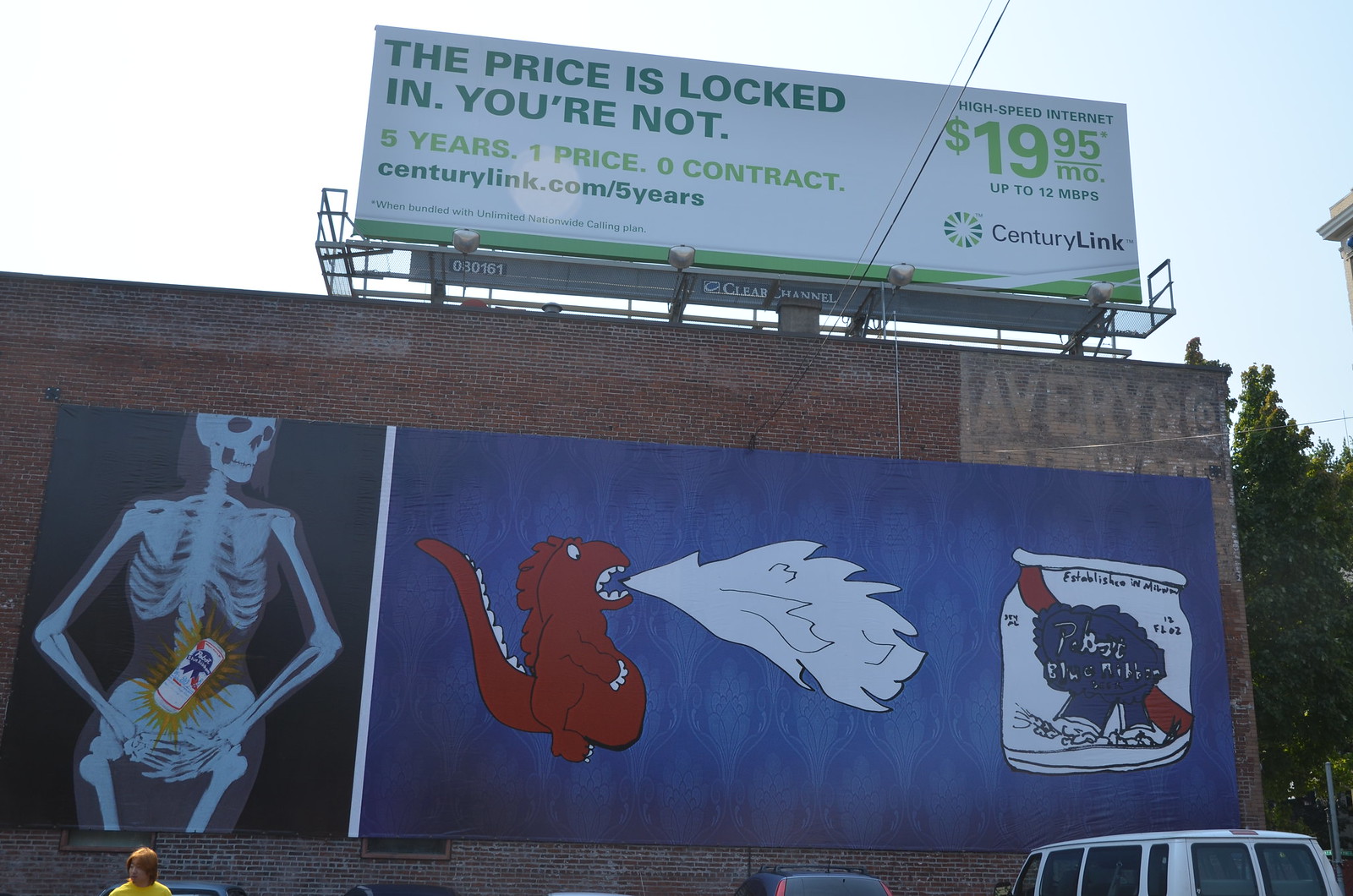This image captures a vibrant urban scene featuring striking street art on the side of a brown brick building. At the bottom of the artwork, there is a character depicted with a visible head and upper torso. This character sports a yellow shirt and has shoulder-length brown hair. Adjacent to the character, we see the roof of a black SUV and the top of a white van adorned with numerous windows.

The building itself is composed of brown bricks and has a billboard positioned at the top. The billboard features a black underbase with green text reading, "The price is locked in, you're not," and an additional line in lighter green text stating, "five years, one price, zero contract, centurylink.com/fiveyears." Below this, the billboard advertises "$19.95 per month, up to 12 Mbps, CenturyLink" in bold text within a white rectangular sign.

The wall art is the centerpiece of the image, depicting a skeleton illustrated in white against a black background. Intriguingly, there is a Pabst Blue Ribbon can placed around the skeleton's stomach area. To the right of the skeleton, a red dinosaur breathes white fire onto another Pabst Blue Ribbon can, painted in its iconic red, white, and blue colors. Completing this eclectic scene, a green tree stands on the far right, with a backdrop of a partly cloudy blue sky enhancing the vividness of the setting.